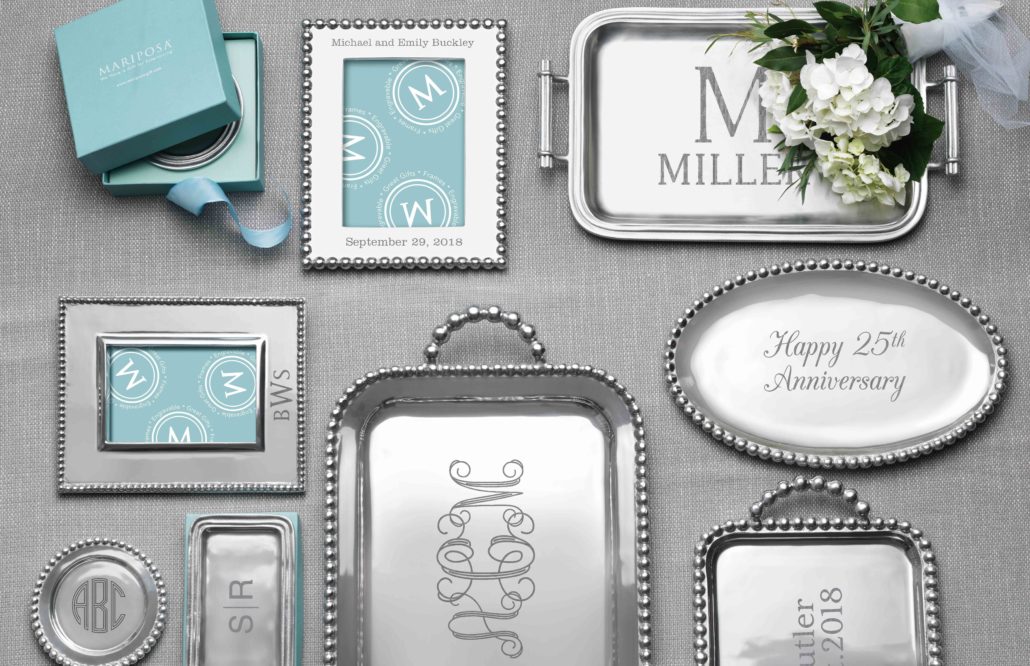An overhead view of personalized silver gifts displayed on a pale gray, metallic-looking fabric surface. The top right features a small wedding bouquet of white flowers with a tulle-wrapped handle. In the top left, an open blue box labeled "Mariposa" reveals a blue ribbon curling out. Nearby, a variety of intricately designed silver items are arranged. This includes a photo frame with a light blue background and an "M" logo, engraved with the initials "BWS." Another larger jeweled-edge photo frame also features the monogram "M" and is engraved with "Michael and Emily Buckley, September 29, 2018." There is a silver coaster with a beaded edge monogrammed "ABC." Among the four different platters, an oval tray reads "Happy 25th Anniversary," and a square tray with rounded corners is inscribed with "SR." Another features the initial "M" followed by "Miller." The shared elegance of these engraved gifts against the unified gray background creates a sophisticated array.